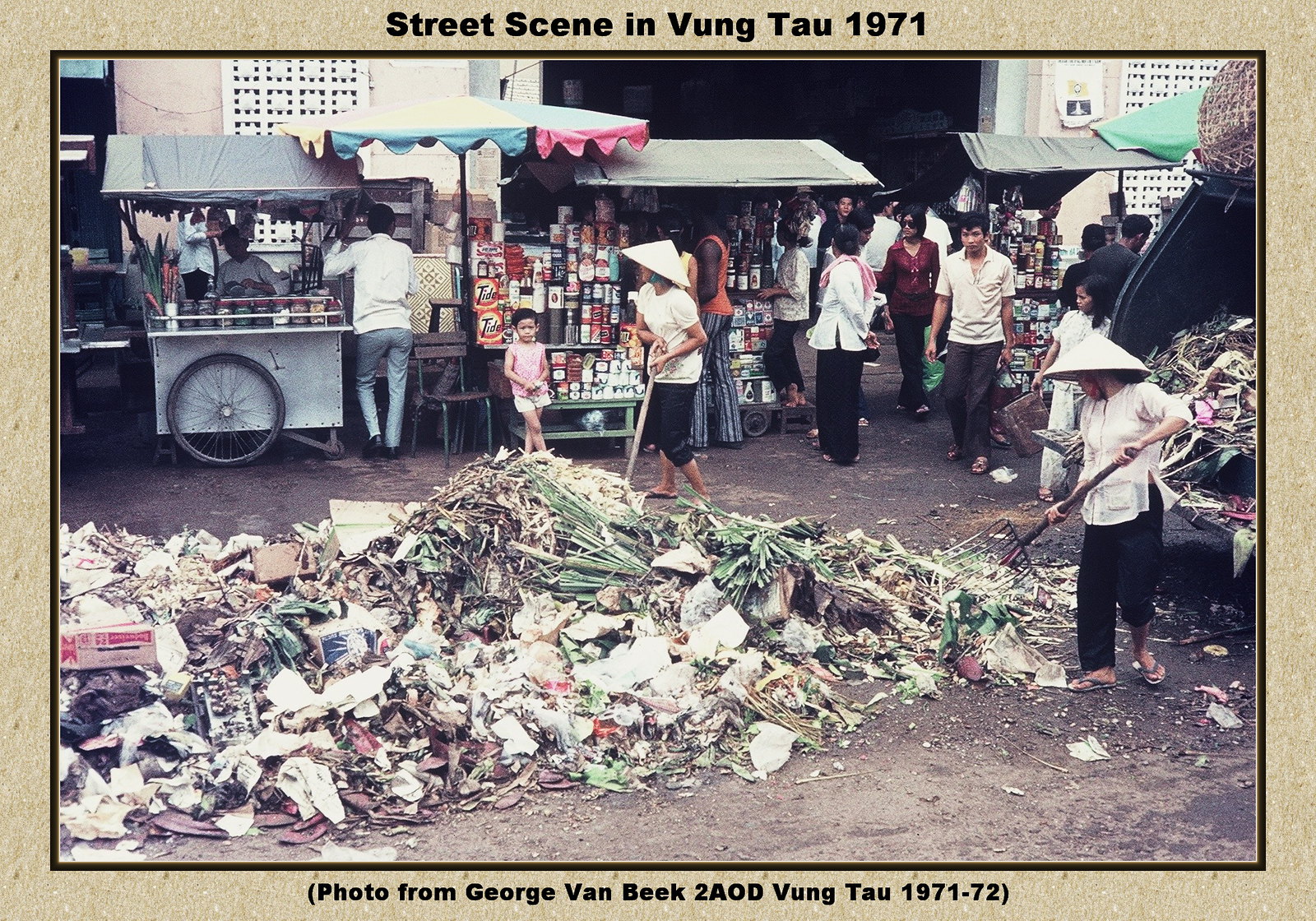The photograph, prominently framed with a tan-colored border and a dark, thinner inner line, captures a lively street scene in Vung Tau, Vietnam, in 1971. At the top of the border, black text reads, "Street scene in Vung Tau, 1971," while the bottom text states, "Photo from George Van Beek to AOD Vung Tau, 1971-72." The image depicts an unpaved street cluttered with various detritus, including grass, trash, and miscellaneous garbage. 

In the heart of the scene, two women are diligently raking the debris into a pile. One of the women uses a pitchfork to scoop the trash into a nearby garbage truck. This truck, already filled with refuse, is parked on the right side of the street. The background reveals an open market atmosphere, with multiple stalls lining the street, selling food, household items, and various other products. Shoppers and pedestrians move about, some stopping at the temporary shops, while others meander through the scene. Beyond the bustling market, the faint outlines of buildings and a large gateway can be seen, anchoring the vibrant activity of the street in its specific locale and time.